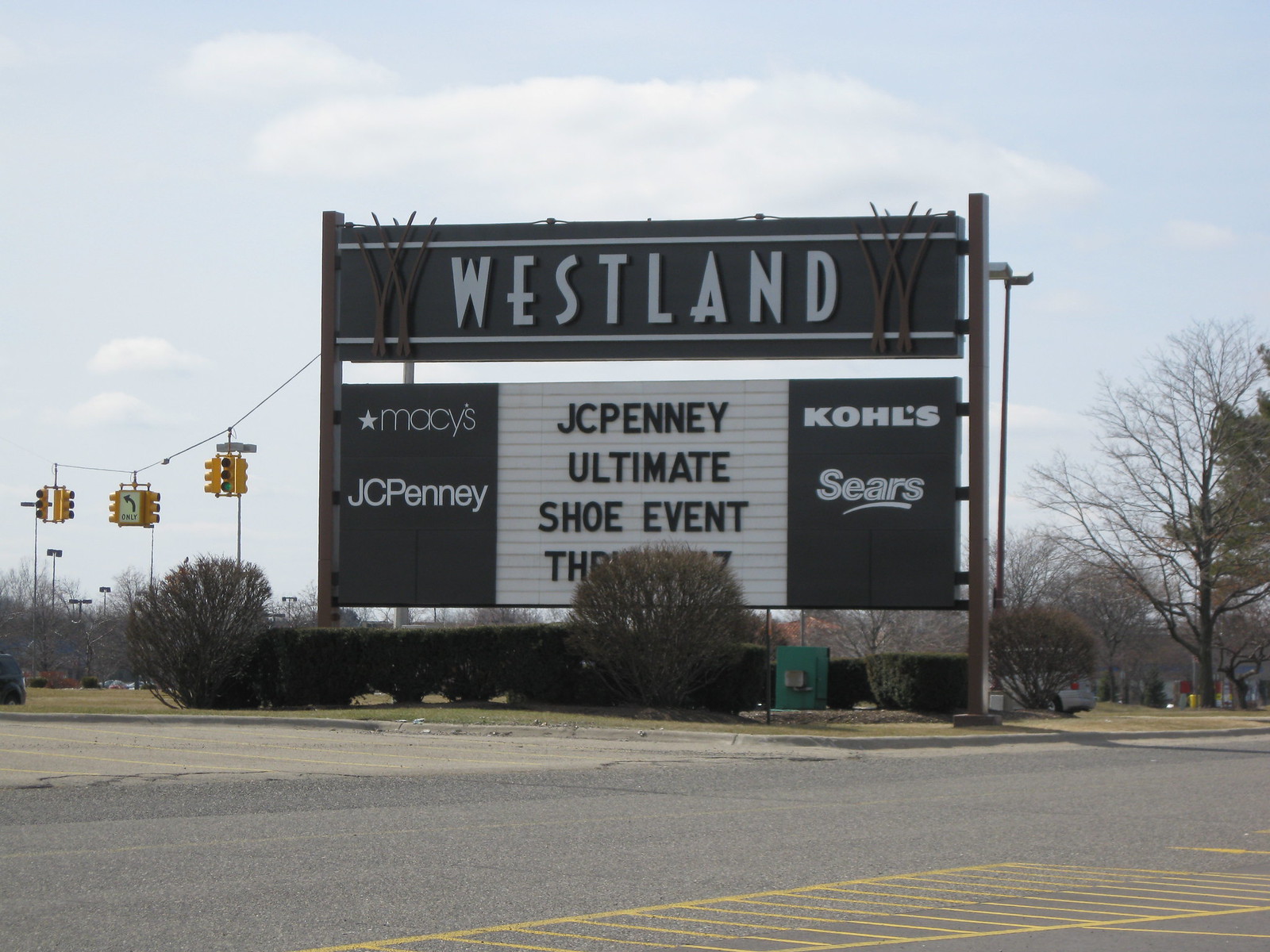A photo captures a bright, sunny day outside, taken from across the road. Prominently featured in the center is a large sign, marking the main entrance to a shopping center named "Westland." The towering sign is mounted on two heavy metal poles, with its top section colored black and adorned with the shopping center's name in bold white letters. Beneath this, the sign is divided into two black panels—one on the left displaying the store names "Macy's" and "JCPenney," and one on the right listing "Kohl's" and "Sears." Nestled in the middle is a white marquee, announcing the "JCPenney Ultimate Shoe Event" in black letters, though the exact dates are obscured by a bush. Lush landscaping with various bushes surrounds the base of the sign, adding a touch of greenery. In the foreground, the entrance to the parking lot is clearly visible, with a well-marked asphalt road featuring a yellow-bordered island in the center. Notably, no cars are present on the road, emphasizing the placid atmosphere of the scene.